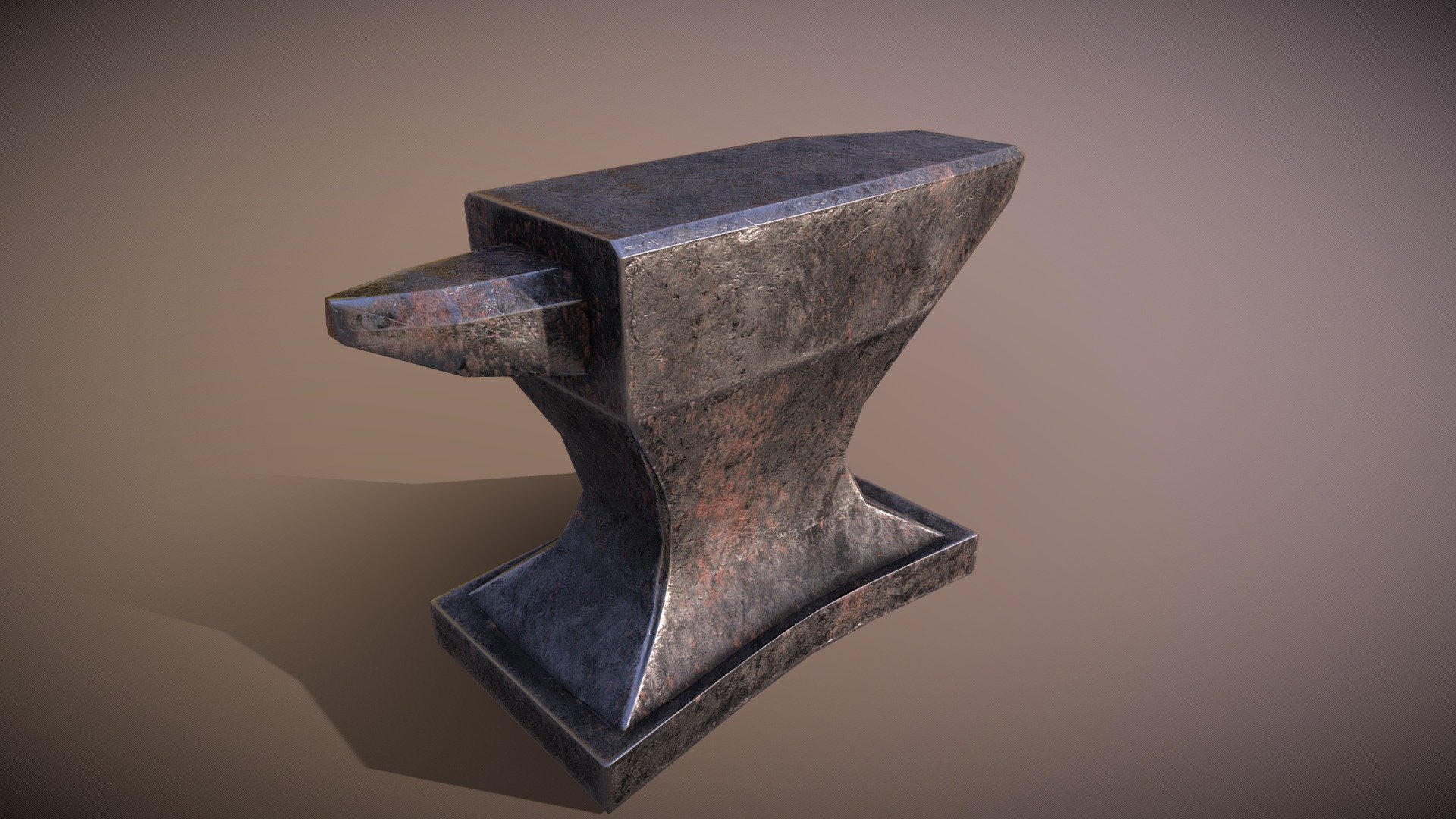The image depicts a detailed 3D rendering of an anvil with an attractive, shiny copper and black, reddish coloration, positioned against a copperish-brown background. The anvil has a flat top and bottom, narrowing in the middle before widening into a rectangular base. Notably, there is a small, horn-like protrusion on the top left side of the anvil. The surface appears worn, indicative of prior use, with visible marks and dents. The anvil is well-lit from the right, casting pronounced shadows to the left, enhancing its realistic and heavy appearance, making it look like a polished display piece suitable for a museum exhibit.